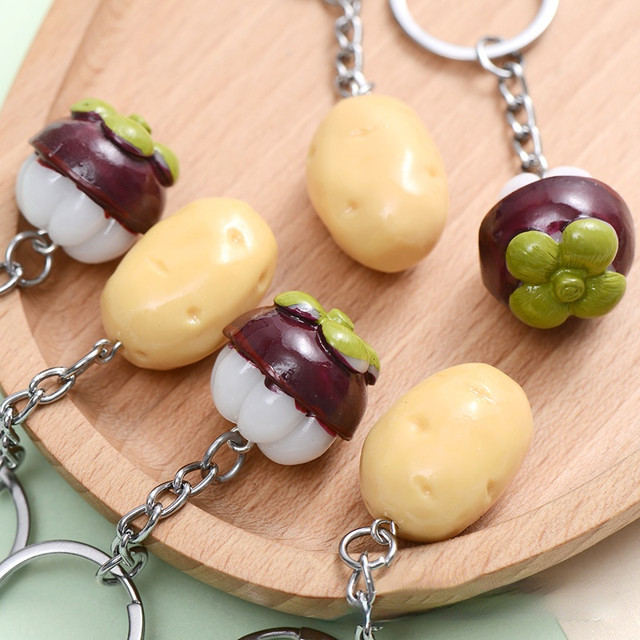The image features a wooden oval cutting board placed atop a two-toned table — half green and half a light blue or white hue. On the board, there are six keychains, each with a miniature vegetable or fruit. Three keychains display small potato replicas, and the other three showcase radish-like figures with green tops and purple-white bodies. The keychains are all connected to silver metal rings, which are meant to attach to keyrings. The scene is shot indoors from a top-down perspective, highlighting the details and arrangement of the keychains.